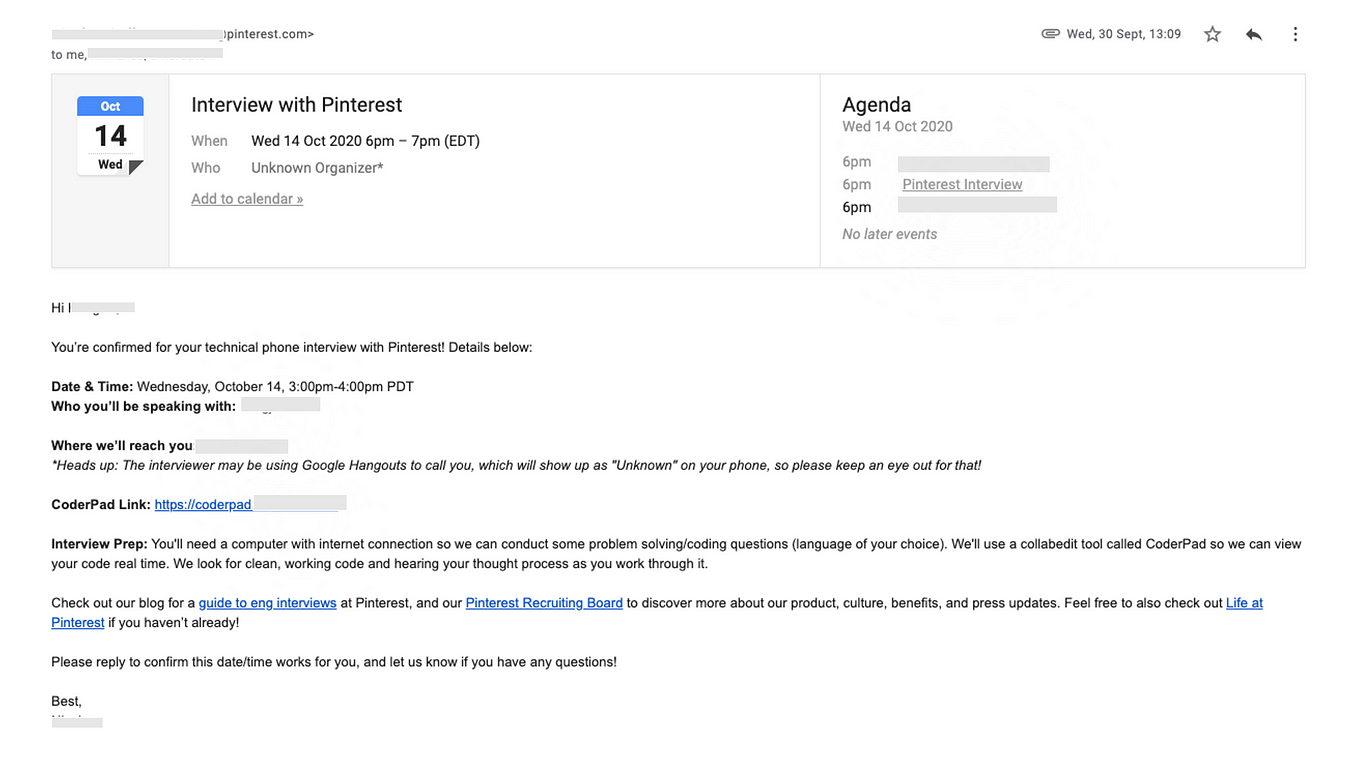**Detailed Caption:**

The image is a screenshot of an email displayed on a white background. The email contains information about a scheduled technical phone interview. On the left side, the date is shown as "Wednesday, 30 September," and the time is "1309." The sender's email address is obscured by a gray line for privacy.

At the top left of the email, there is a small gray box with a square inside it. The top of this square features the word "October" in white font against a blue background, and below it, in large bold numbers, "14" indicating the date, with "WED" for Wednesday written underneath. To the right of this, the text reads "Interview with Pinterest," detailing the specific date and time as "Wednesday, 14 October 2020, 6 to 7 p.m. EDT," along with an agenda marked with the same date and additional details that are redacted for privacy.

In the body of the email, the salutation "Hi" is addressed to the recipient whose name is blotted out. The email confirms the technical phone interview with Pinterest, specifying: 

- **Date and Time:** Wednesday, October 14th, 3 p.m. to 4 p.m. PDT
- **Interviewer and Contact Details:** Redacted with gray lines

A note advises the recipient that the interviewer might use Google Hangouts, which will display as an unknown number on their phone. There is a "coder pad" link included, parts of which are redacted.

The email outlines the interview preparation requirements, emphasizing the need for a computer with an internet connection to solve coding questions in the recipient's choice of programming language using a collaborative tool called CoderPad. It stresses the importance of providing clean, working code and articulating the thought process during the interview.

The email concludes with a request for the recipient to confirm the date and time, offering assistance for any questions they might have, and is signed off with "Best," followed by the sender's name, which is also blotted out for privacy.